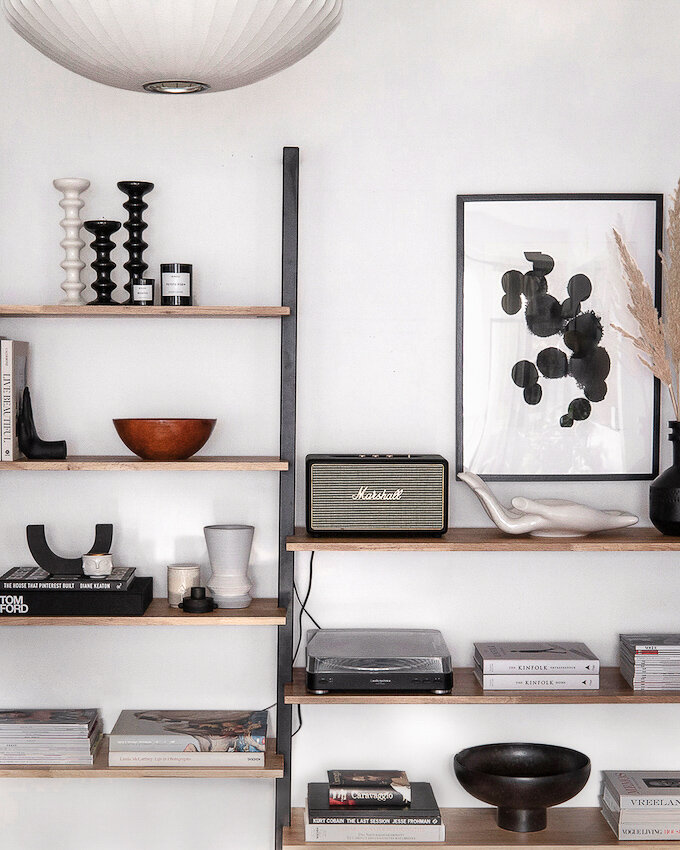This image captures a detailed view of a modern living room's dual-unit shelf system, characterized by black metal frames and medium brown wooden shelves, all mounted on a pristine white wall. On the tallest unit to the left, the top shelf features three modern textured candlesticks—one white and two black—alongside two candles. The second shelf holds a decorative brown bowl and a book positioned by a bookend. Below this, the third shelf displays an arrangement of vases and additional books. The bottom shelf houses a collection of neatly arranged books.

To the right, the slightly lower unit starts with a Marshall stereo system, identified by its vintage design and cursive branding. Next to it, a white ceramic hand sculpture, with fingers spread out gracefully, stands under a black-and-white abstract painting framed in black. Below the stereo, an additional electronic unit, presumably a vintage turntable for vinyl records, is positioned beside a set of white-covered books. The lowest shelf of this unit has more books, with a large decorative black bowl with a thin cylindrical base centrally placed, flanked by additional books on either side.

Enhancing the overall aesthetic, a white glass light fixture is discernible hanging from the ceiling, further illuminating the meticulously arranged and stylishly clutter-free display. This setting exemplifies a blend of modern and vintage elements, achieving a sophisticated yet homely atmosphere.